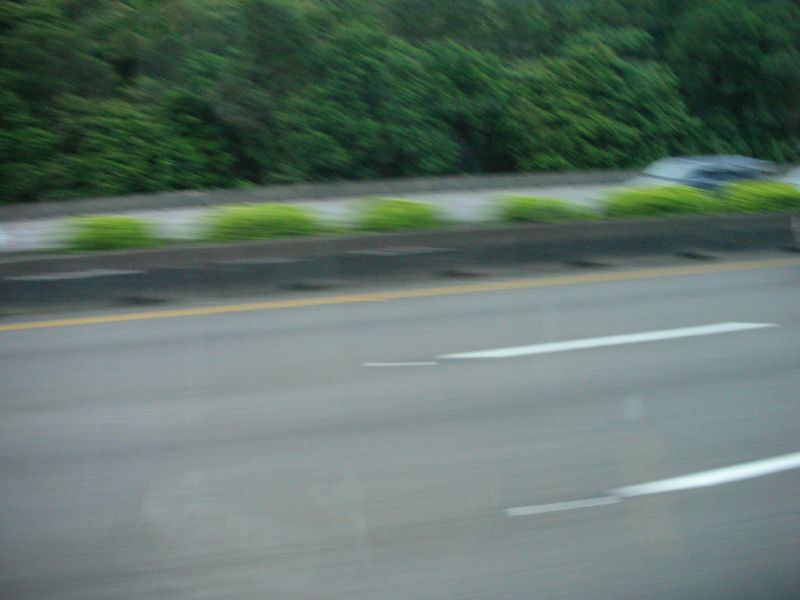Speeding down the highway, this dynamic photograph captures the essence of rapid motion from the perspective of a car traveling north-south. The image is intensely blurred, emphasizing the swift pace. The scene depicts a three-lane highway divided by a central strip adorned with a guardrail and patches of shrubbery. On the opposite side of the highway, an indistinct car whirs by, barely recognizable due to the blur. The background reveals glimpses of trees and foliage, further obscured by the speed. 

Every element in the photograph—from the blurred lanes to the fleeting streaks of passing vehicles—conveys the sensation of high-velocity travel, encapsulating the exhilarating experience of racing down a busy freeway.